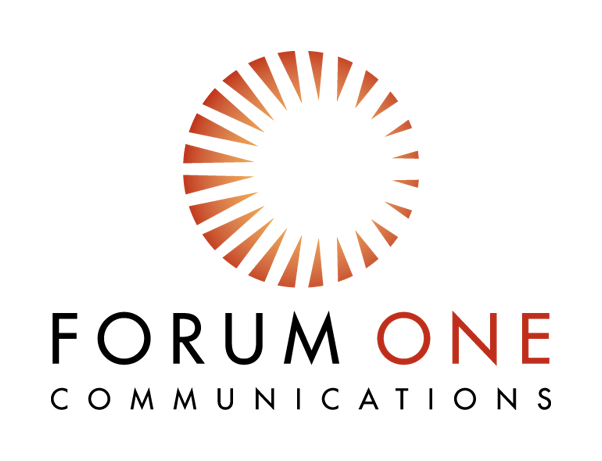The digital image features the logo of the company Forum One Communications. The logo, centered on a plain white background, showcases a circular design composed of variously sized red triangles forming a ring with a hollow center, reminiscent of a stylized sun. Below this intricate emblem, the company name is displayed with "Forum" and "One" in larger black letters, and "One" in a striking red color. The word "Communications" appears beneath in much smaller black letters, precisely aligned so the 'C' in "Communications" lines up with the 'F' in "Forum" and the 'S' aligns with the 'E' in "One," creating a balanced and cohesive visual arrangement.